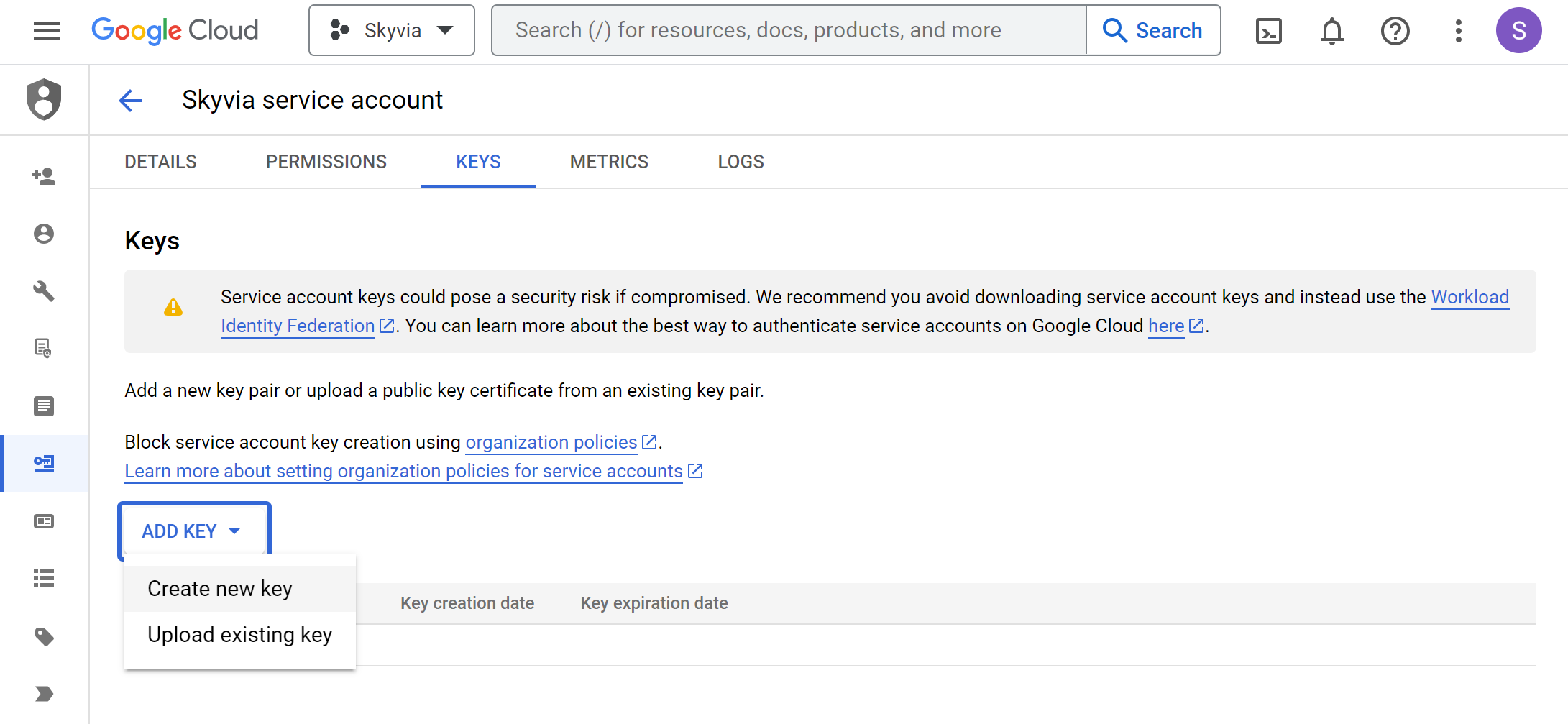This image is a detailed screenshot of the Google Cloud console interface. The background is white, ensuring clarity and focus on the interface components. 

### Header Area
- **Top Left Corner**: The header features the text "Google Cloud" where "Google" is stylized in the company logo colors with a blue "G," red "o," yellow "o," blue lowercase "g," red "l," and green "e." The word "Cloud" appears in gray.
- **Menu Icon**: To the left of the "Google Cloud" text, there are three horizontal gray lines representing a dropdown menu.

### Top Center
- **Search Box**: Centered in the header is a light gray search box with the placeholder text "Search for resources, docs, products, and more."

### Top Right Corner
- **Account Icon**: On the far right, there is a purple circle with a white letter "S" in the center.

### Left Sidebar
- **User Account and Navigation**: The left sidebar displays "Skyvia Service Account" with a sub-menu including "Details," "Permissions," "Keys," "Metrics," and "Logs." 
- **Icons**: The sidebar features various icons such as a gray account icon, a wrench (likely for settings), and document icons.

### Main Content Area
- **Keys Section**: Beneath the sub-menu, the "Keys" section is highlighted.
  - **Warning Message**: A gray rectangle contains a yellow triangle with a white exclamation mark, signaling a warning. The text reads: "Service account keys could pose a security risk if compromised. We recommend you avoid downloading service account keys and instead use [Workload Identity Federation](external link)." The recommendation is hyperlinked and written in blue with an external link icon.
  - **Additional Information**: Following the warning, there's a note stating: "You can learn more about the best way to authenticate service accounts on Google [here](external link)." "Here" is a blue, underlined hyperlink with an external link icon.

The detailed layout efficiently guides the user through the Google Cloud console's features, emphasizing security measures and navigation options.